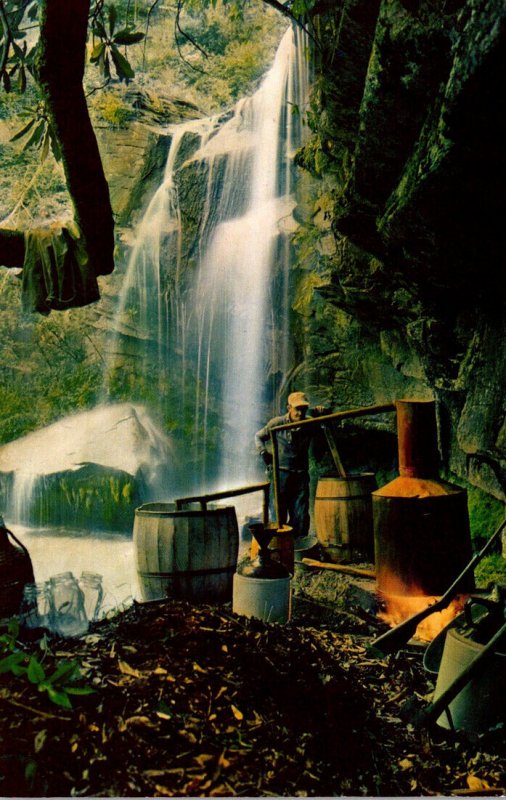The image features a picturesque outdoor scene centered around a waterfall cascading from a lush, grassy, and shrub-filled area on the left, descending towards a rocky cliff on the right. In the lower right corner, there's a rusted metal stove with a rounded, tapered roof and a flame underneath it, evoking a wheelbarrow-like appearance. Adjacent to the stove stands a man dressed in a brown hat, blue shirt, and blue jeans. Surrounding the man are several wooden barrels and a contraption suggesting a whiskey still, given the array of glass jars and bottles nearby. A large pole protrudes from one barrel, connecting via a pipe to a smaller stove and leading to another wooden barrel. This setup is situated on a mulchy ground, with patches of green grass interspersed around it. The image is taken in bright, clear daylight, bringing out the vivid colors of the natural landscape and the clarity of the scene.